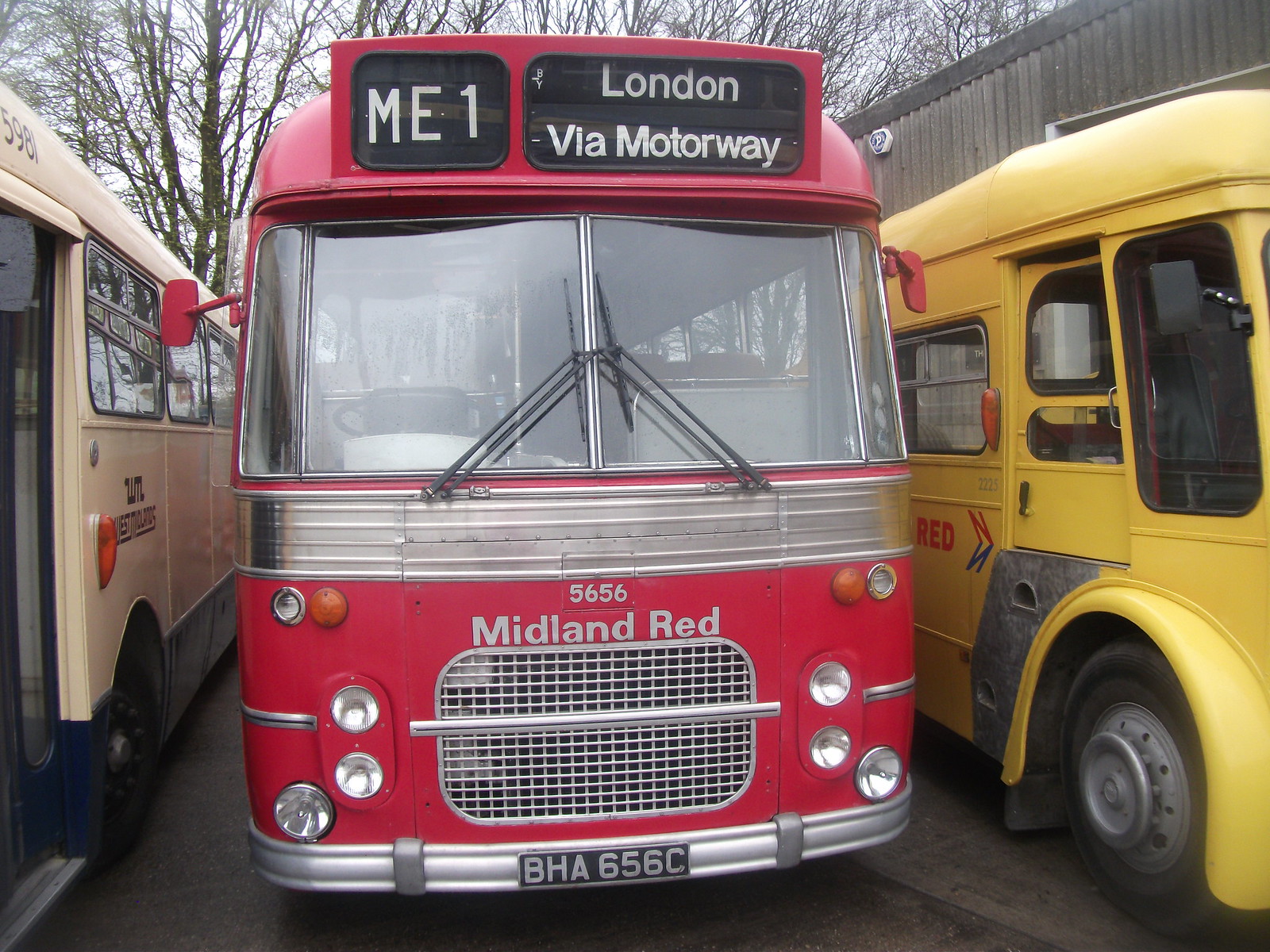The photograph captures a vivid scene featuring a classic red bus prominently set in an outdoor parking lot, flanked by a yellow bus on its right and a white bus with a blue stripe on its left. This red bus, reminiscent of mid-20th-century designs, stands out with its various details. At the top of the bus, an informational sign reads "ME1" on the left and "London via motorway" to the right. Just below this sign, the bus's large, clear front windshield is divided into two square panes equipped with windshield wipers. Below the windshield is a silver border that's part of the overall robust front design. The bus's front end displays the text "5656 Midland Red" above a front grille, complemented by a license plate that reads "BHA 656C." The front of the bus also features four headlights and additional running or emergency lights. The scene is further enriched by the natural lighting and a backdrop of trees and branches, adding a scenic element to this nostalgic portrayal of classic transportation.